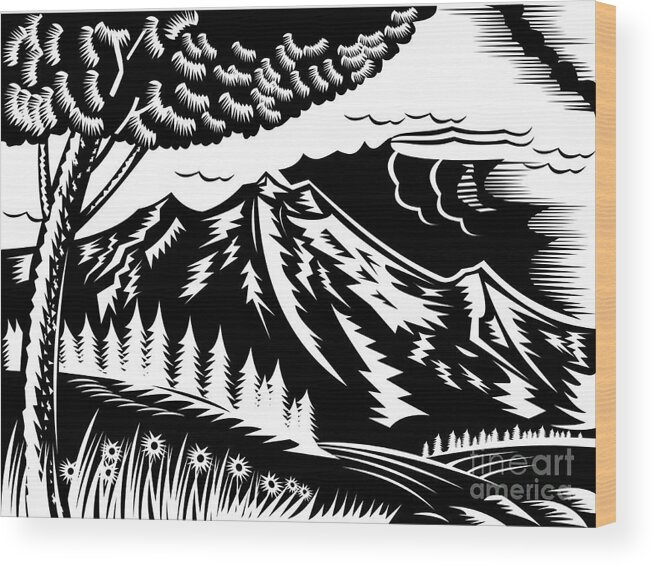This detailed black and white artwork, created by Fine Art America and displayed on a wooden canvas, presents a striking mountainscape. The foreground features an intricate arrangement of white flowers and grass, contrasted against a darker background due to the use of negative space. To the left, a prominent tree stretches from the bottom to the top of the image, its upper sections extending beyond the canvas. The central portion of the artwork is dominated by a majestic, rocky mountain, with approximately fifteen pine trees ascending its slope. Above the mountain, an expanse of clouds fills the sky, darker and stormier to the right, transitioning to calmer, whiter formations on the left. The label "Fine Art America" is visible in white text at the bottom right of the canvas.